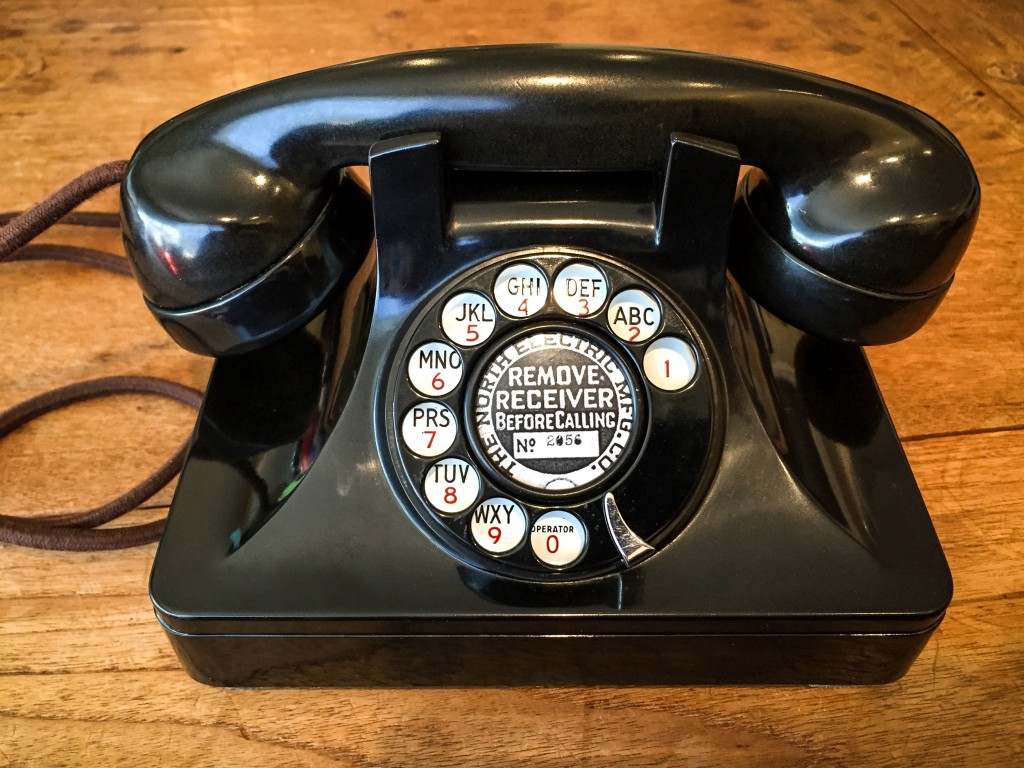This is a detailed photograph of a vintage black rotary phone placed on a brown wooden surface. The phone features a circular rotary dial prominently in the middle, which displays numbers 0 through 9, each paired with three corresponding black letters. In the center of the dial, within a small circular area, text reads "The North Electric MFG Co., remove receiver before calling number 2056." A barbell-shaped receiver handle for listening and speaking is attached to the phone along with a brown, non-stretchable cable. The phone’s shiny black surface contrasts with the brown hue of the wooden parquet table. Additionally, a small metallic piece on the side of the phone serves as a finger stop.